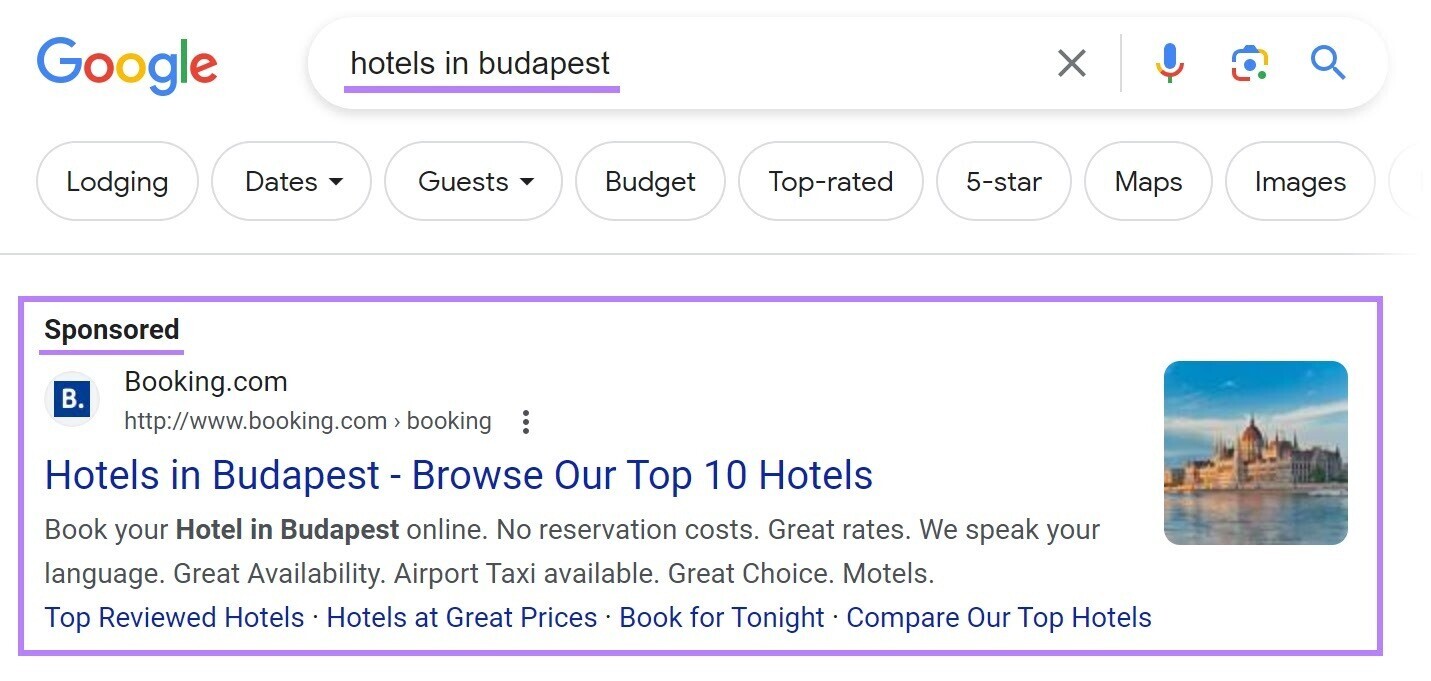The screenshot features a white background with the Google logo displayed in its signature multi-colored font in the upper left corner. Adjacent to the logo, there is a long, horizontal, oval-shaped search bar. Inside the search bar, the query "Hotels in Budapest" is written in black text and underlined with a purple line. On the right side of the search bar, there are icons arranged sequentially: a gray "X," a microphone, a square, and a magnifying glass.

Below the search bar, a series of buttons are visible: "Lodging," "Dates" (accompanied by a drop-down arrow), "Guests" (also with a drop-down arrow), "Budget," "Top Rated," "5 Star," "Maps," and "Images." Another partially visible button is noted at the edge of the oval area, all underlined with a thin gray line.

Further down, the layout includes a highlighted rectangle outlined in purple. In the upper left corner of this rectangle, in bold black text underlined in purple, it reads "Sponsored." Directly below this is the Booking.com logo, with the accompanying text "Booking.com" to its right. Beneath the logo, the Booking.com website URL is displayed.

To the right side of the rectangle, there is a square image depicting a scenic view of a castle-like structure with a body of water in the foreground and a blue sky above.

Returning to the left section of the rectangle, there is a blue header "Hotels in Budapest - Browse our top 10 hotels." Following this, black text reads: "Book your hotel in Budapest online. No reservation costs, great rates, we speak your language, great availability, airport taxi available, great choice, motels."

The final portion includes blue hyperlinks stating: "Top reviewed hotels," "Hotels at great prices," "Book for tonight," and "Compare our top hotels."